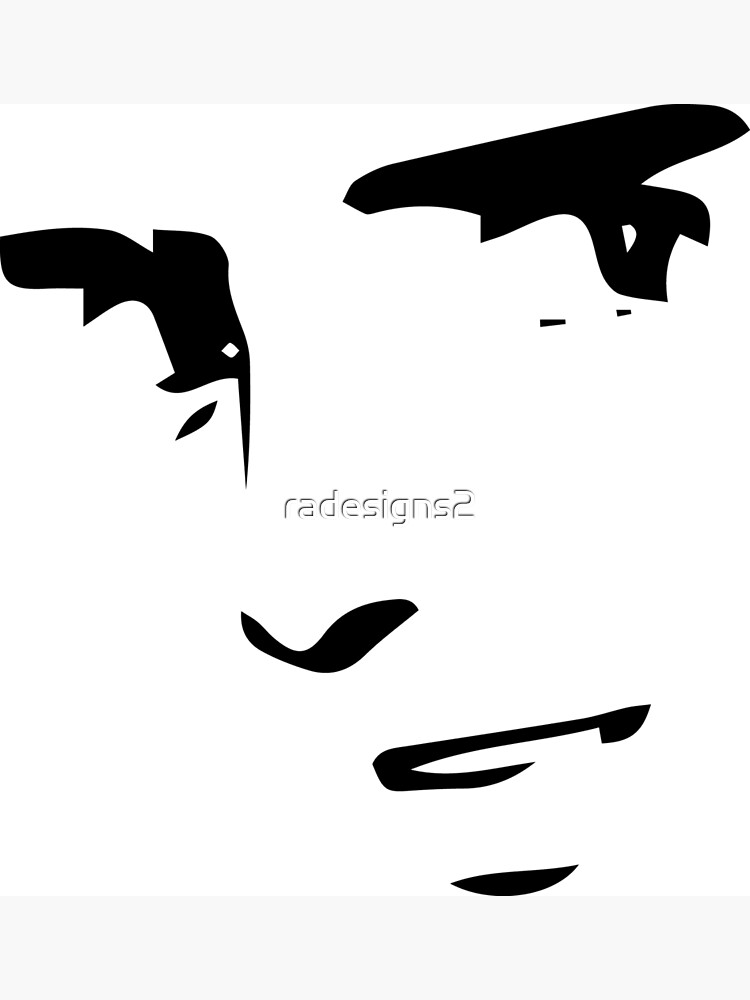The poster, set against a stark white background with a small strip of pale gray at the top, showcases an abstract rendition of a face created with solid black ink blots. These blots form distinct facial features without defining the face's width or height, giving it a minimalist and mysterious aesthetic. The eyes and eyebrows are depicted with dark blotches, while a subtle line extends from the right eye down, representing the bridge of the nose. Approximately an inch below, a swirl indicates the nose tip. Beneath this, a sideways hook symbolizes the mouth, and a dash below it suggests the chin. The entire face appears to be turned slightly to the right. In the midst of these features, centrally located, are the words "RADESIGNS2" written in white lettering. This stylized portrayal forms the only details on the otherwise empty white expanse, presenting a strikingly modern and avant-garde visual.